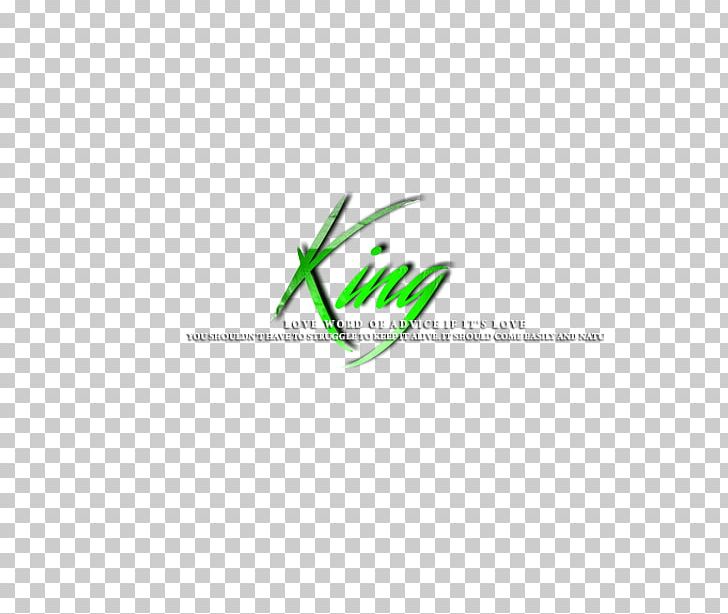The image, likely an advertisement for the company King, features a checkered background composed of numerous small gray and white squares. At the center, the word "King" is prominently displayed in a highly stylized, flourishy, chic font with different shades of green, making it stand out. Below "King," in much smaller and difficult-to-read text, the image includes a phrase that seems to read "love word of advice, if it's love, you shouldn't have to struggle to keep it, it should come naturally." The white color of this secondary text blends into the checkered background, making it challenging to decipher.